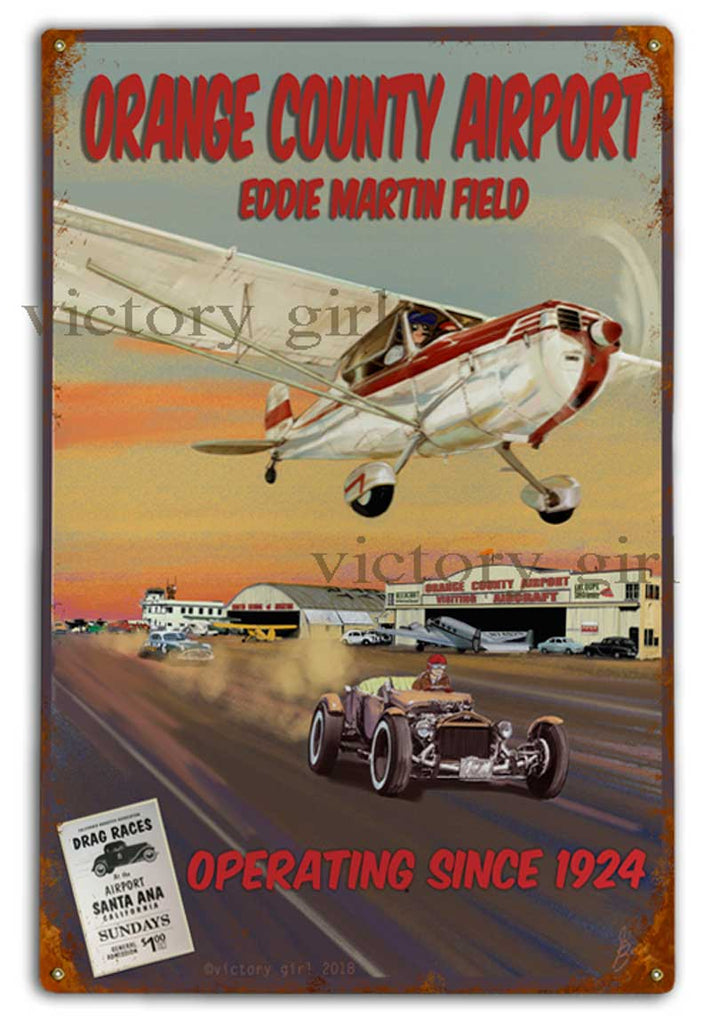The image depicts a vintage tin sign with distinct signs of age, such as rusted red distressed edges and gold eyelet studs in each corner. The central image showcases a dynamic scene of a racing speedway set against an airport backdrop. Across the top in bold red text, it reads "Orange County Airport, Eddie Martin Field," referencing the well-known locale. Just below, a striking painting-style depiction captures a red and white propeller plane soaring in mid-flight.

Beneath the airborne plane, a gray roadway bustles with old-style race cars hurtling down the speedway. In the foreground, a particularly eye-catching black and silver metallic race car with white seats is driven by a man donning goggles and a red hat. This action-packed scene is accentuated by red text towards the bottom, stating "Operating Since 1924." To the left of this text, a smaller white and black flyer advertises "Drag Races, Airport, Santa Ana, Sundays, $1," featuring a side profile of a vintage black car.

In the distant background, a couple of buildings reminiscent of garages are visible, adding depth to the image. The skyline is artistically rendered in an ombre palette of yellow, orange, and blue, suggestive of a sunset. A faint watermark at the bottom reads "Copyright Victory Girl 2016," while a larger gray watermark stating "Victory Girl" appears twice at varying angles over the sign. The entire composition reflects the charm and vibrancy of an old-timey racing era, effectively conveying the historical significance and spirited atmosphere of Orange County Airport.